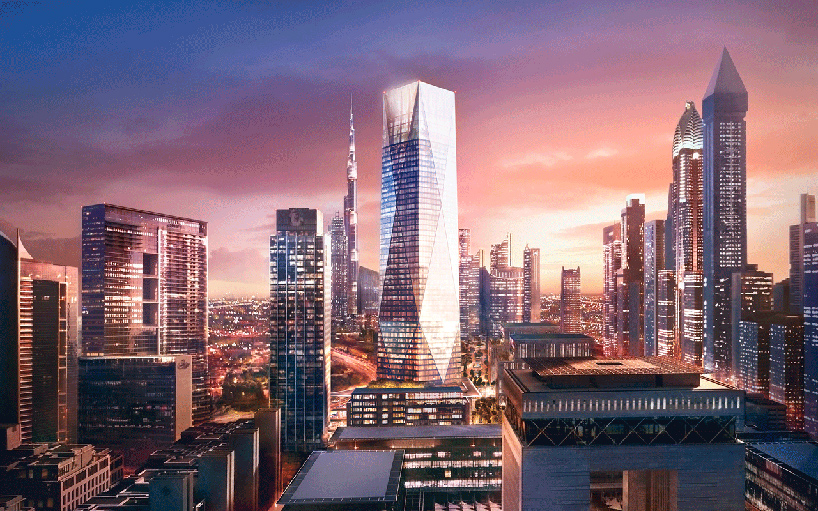A vibrant cityscape is displayed at twilight, featuring an array of towering skyscrapers set against a stunning, multi-hued sky. The skyline is dominated by a central rectangular skyscraper that gleams with reflected sunlight. Next to it on the right stands a thin, spiky building of similar height, while the left features a shorter building with a more geometric pattern. Further to the right, there are two taller, pointed skyscrapers illuminating the scene with their lit windows. The sky transitions beautifully from deep blue to purple, to a reddish-orange gradient with hints of white at the horizon where the sun is setting. Below, a mix of smaller buildings and roadways are visible, with additional lights scattered across distant rolling hills. The clouds add texture to the sky, enhancing the overall picturesque quality of this urban twilight vista.